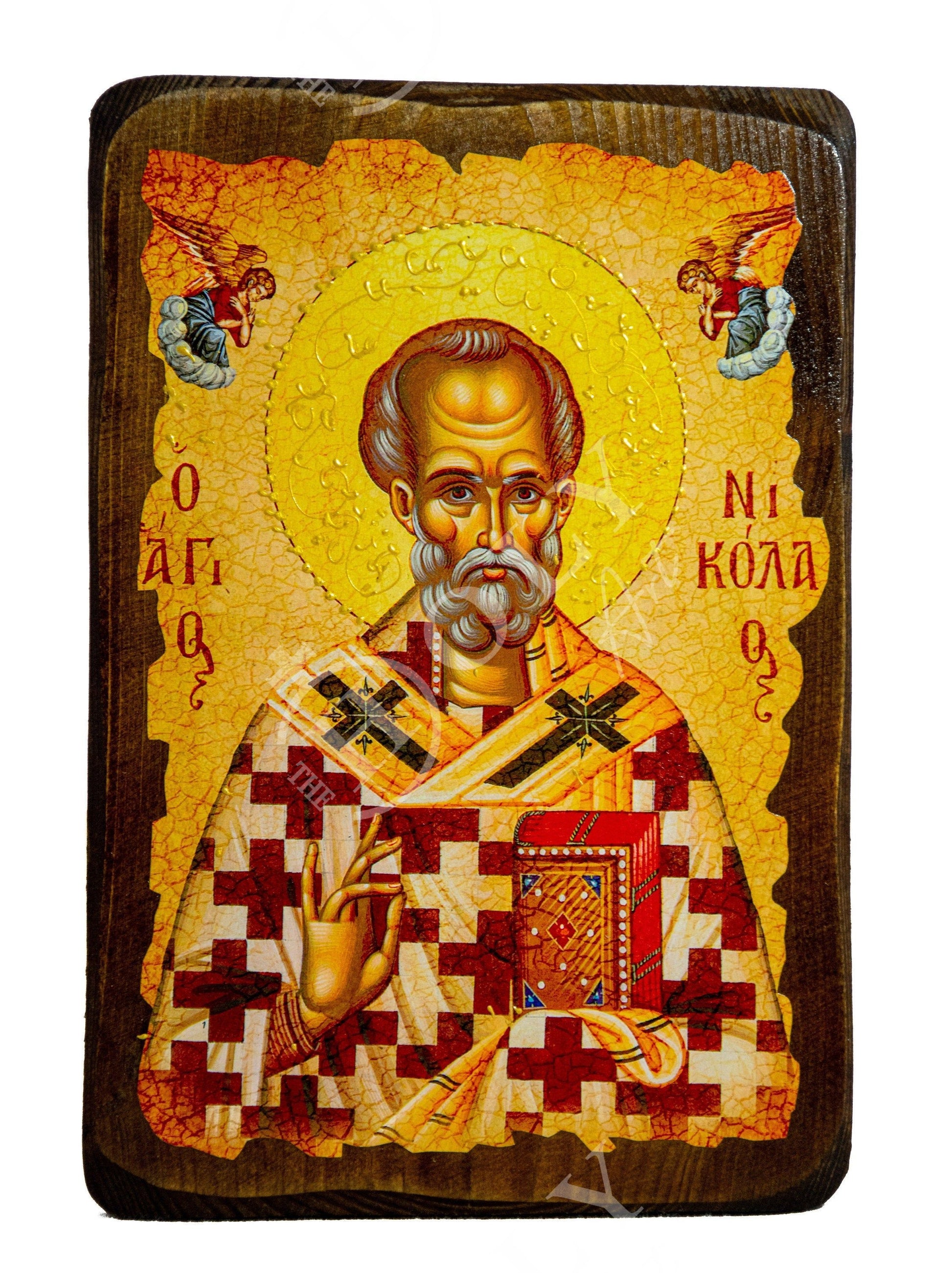This image is a detailed color illustration of a religious figure, likely a saint, set on a wooden-type plaque with rough edges around it. The central figure is an aged man with a gray beard and a balding head, adorned with a halo, marking his saintly or holy status. He wears Roman Catholic-style robes, elaborately decorated with a pattern of red and white crosses. A yellow shawl drapes over his shoulders, featuring two prominent black crosses.

In one hand, he holds a book, possibly a holy text or a deck of tarot cards, while his other hand is raised, with his fourth finger and thumb touching, in a gesture of blessing or benediction. Above the saint, in the top corners of the plaque, two angels with wings are depicted in a prayerful stance. The angels are dressed in red tops and blue skirts, adding an additional layer of sacred symbolism to the scene.